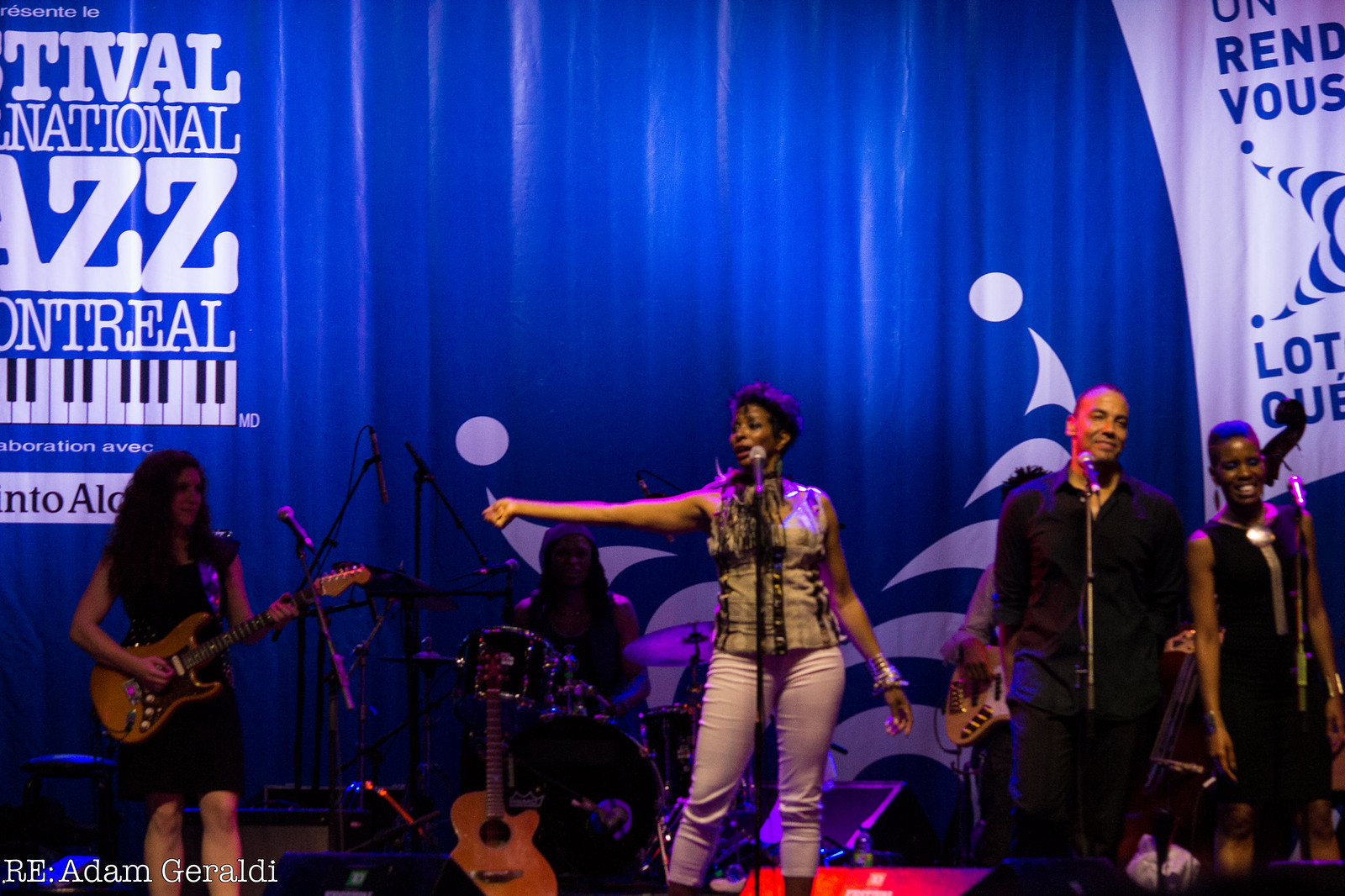The photograph captures a vibrant live performance at the Festival International de Jazz de Montreal, as indicated by the blue curtain backdrop that displays the festival's name alongside a keyboard graphic and a partially visible logo. The credit in the lower left corner attributes the photo to Adam Giraldi. On stage, there are six performers: three vocalists, including an African American woman with short hair in a sleeveless top and brown pants positioned in the center, another female vocalist, and a male vocalist. To the left, a woman guitarist stands with another guitarist nearby. The drum player is positioned towards the back, with an extra guitar propped up on the drum set. The stage's lively atmosphere is captured perfectly, showcasing the energy and dynamism of the jazz festival.